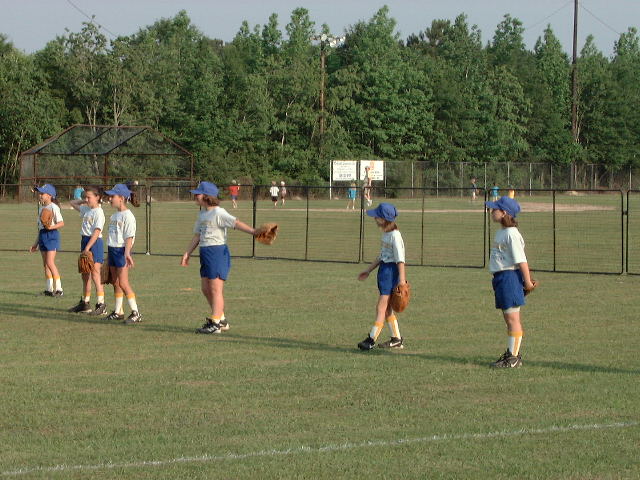In the image, a group of six female baseball players are captured on a grassy baseball field. They are all wearing matching blue shorts that reach their knees and white crewneck shirts, which appear to have some yellow lettering on them, though the text is indistinct due to the distance. Most of the players are sporting blue baseball caps, with the exception of one. Each player has a baseball glove, indicating they are ready for the game. The scene includes a black fence behind the players, and beyond the fence, other children are seen milling around on the field. In the far background, a dense line of pine trees forms a miniature forest, adding to the natural scenery. There also appears to be a disused greenhouse or some structure near the tree line.